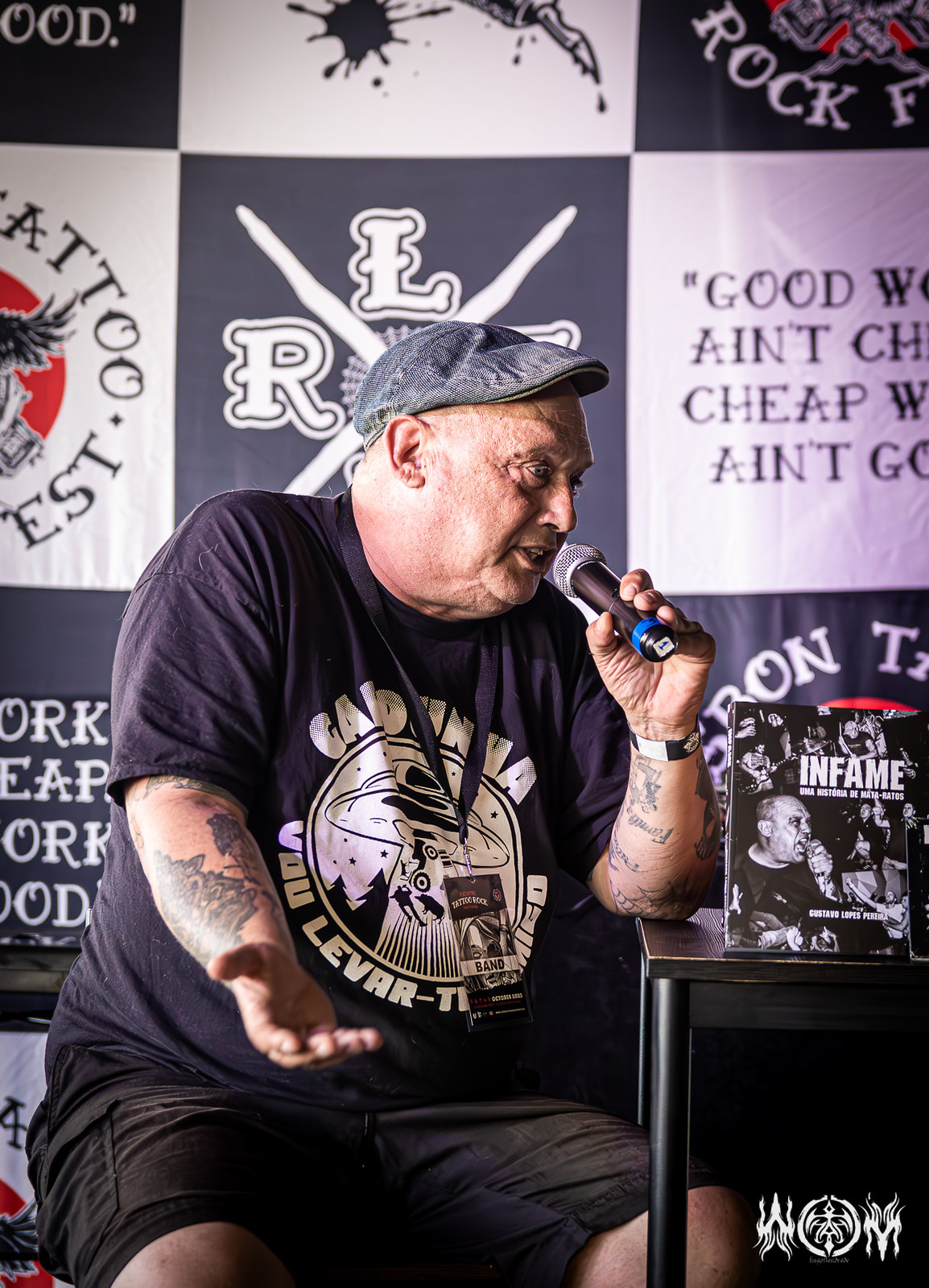In the photograph, an elderly man, likely in his 60s, is captured mid-explanation while seated. He holds a microphone in his left hand, with his right hand outstretched as if emphasizing a point. He is dressed in a distinctive small, bluish blue jean hat and a black t-shirt featuring a somewhat obscured, wrinkled circular logo that appears to be a cartoon spaceship beaming something up, accompanied by some text at the top and bottom. A black lanyard further obscures the logo. The man is also wearing black shorts. 

Adjacent to him on a black table is a book with a predominantly black cover that reads "In Fame" in white text, possibly depicting someone singing alongside a band image. The book appears to be thin and small. Behind the man, a large banner decorated with black and white checkerboard patterns and various logos, some resembling those of metal bands or tattoo parlors, serves as the backdrop. One discernible text on the backdrop reads, "Good work ain't cheap, cheap work ain't good," adding to the environment's eclectic vibe.